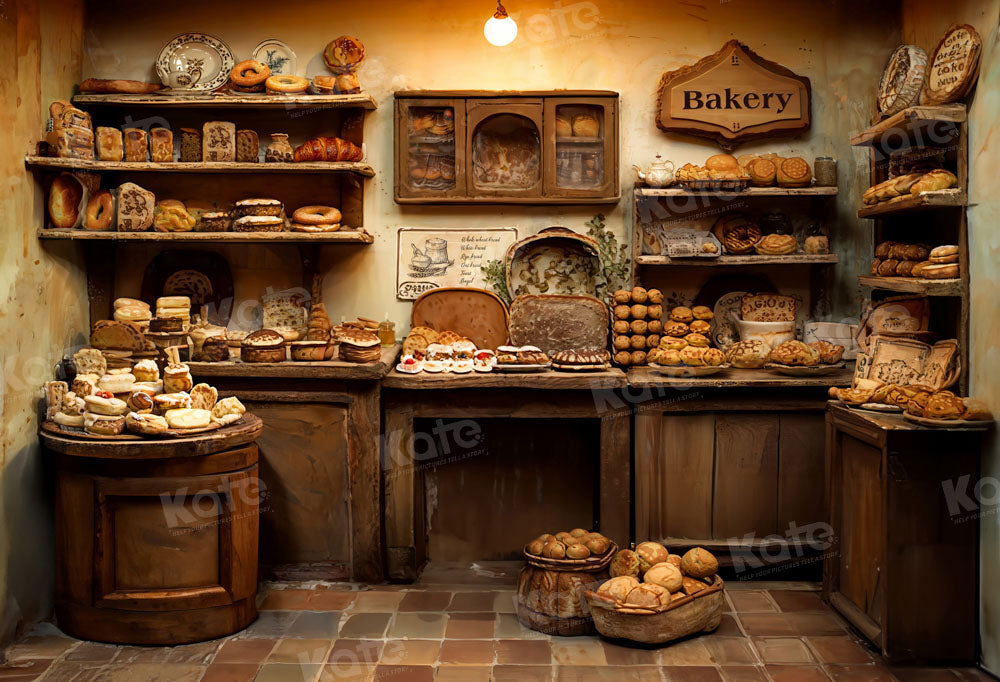This detailed image captures a rustic, old-fashioned bakery with a warm, inviting ambiance. The scene features a variety of earthy browns and yellows, suggesting aged wood and stained stucco walls with a swirling mix of beige and off-white tones. The floor is a patchwork of large, earth-toned tiles interspersed with bits of gray and blue grout. Wooden shelves line the back and right walls, laden with an assortment of baked goods including a variety of breads, rolls, cakes, and pastries. On the left, there is a round table—barrel-shaped—that also holds an array of baked items. At the top right, a wooden sign spells out "bakery," reinforcing the vintage charm. Two bread-filled baskets rest on the floor, adding to the sense of abundance. The cabinetry beneath the shelves is also wooden, although the contents are obscured. A hanging light illuminates the space, enhancing its cozy, old-timey feel. It's notable that the name 'Kate' is monogrammed repeatedly in faded light letters across the image, indicating it is a copyrighted photo.